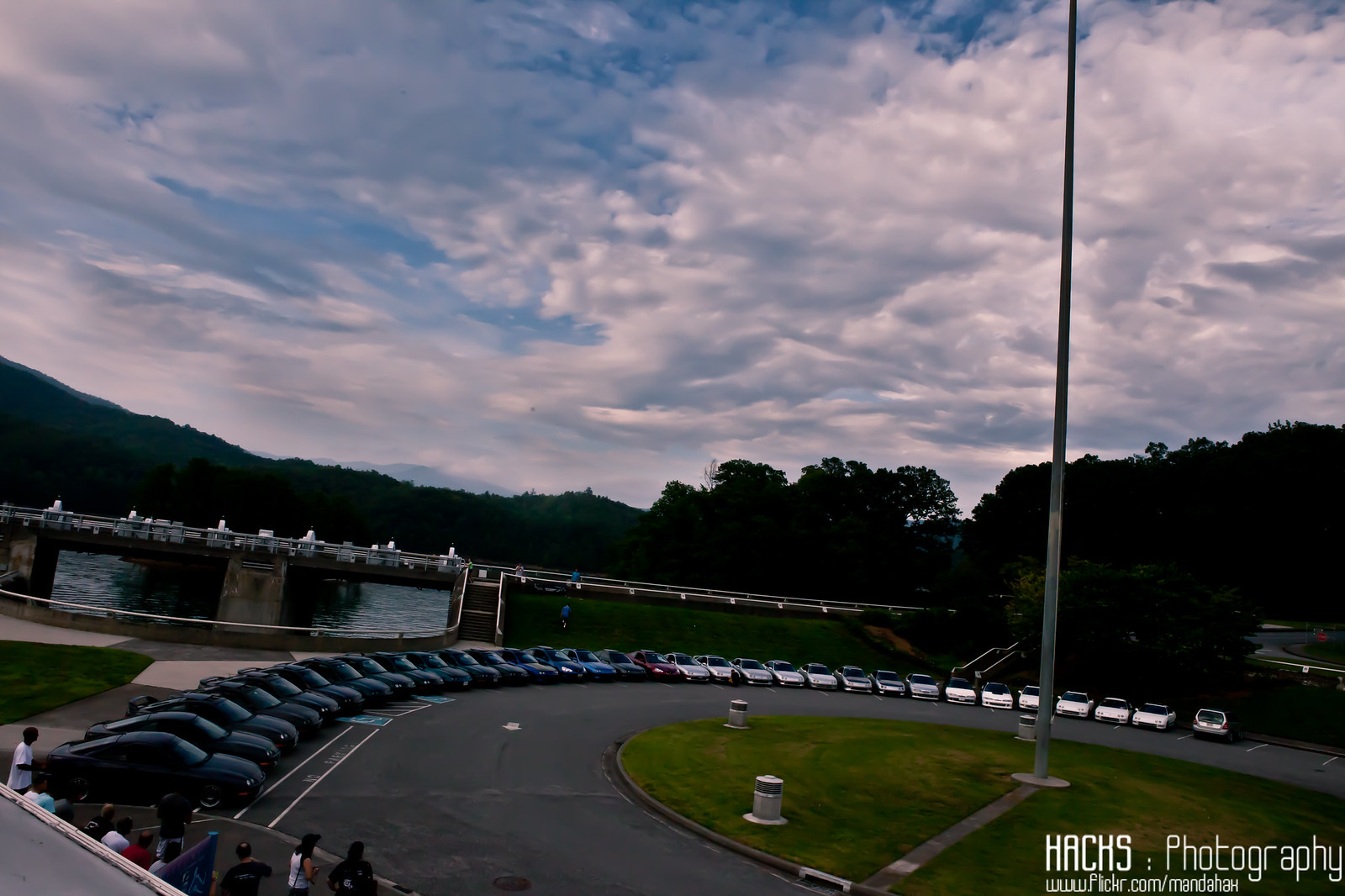This outdoor photograph showcases a circular parking lot surrounded by an asphalt path. The centerpiece of the lot is a large circle of green grass with a tall pole, likely a flagpole, though the top is beyond the photograph's frame. Along the curb of the lot, an array of cars is meticulously arranged, predominantly consisting of identical black sports cars, interspersed with some lighter blue, red, and white cars, emphasizing a purposeful artistic layout. The lot is bordered by a sidewalk and some people are gathered in the lower-left corner, possibly standing or seated. In the backdrop, there's a hill to the left, and several trees frame a set of one-story buildings with large, possibly garage doors that appear open, giving a see-through impression. Above, the sky is a mix of blue and thick white clouds, denser on the right side. The overall lighting is dim, suggesting an overcast day. In the bottom right corner of the photo, text reading "HACHS Photography" along with a web address is visible.